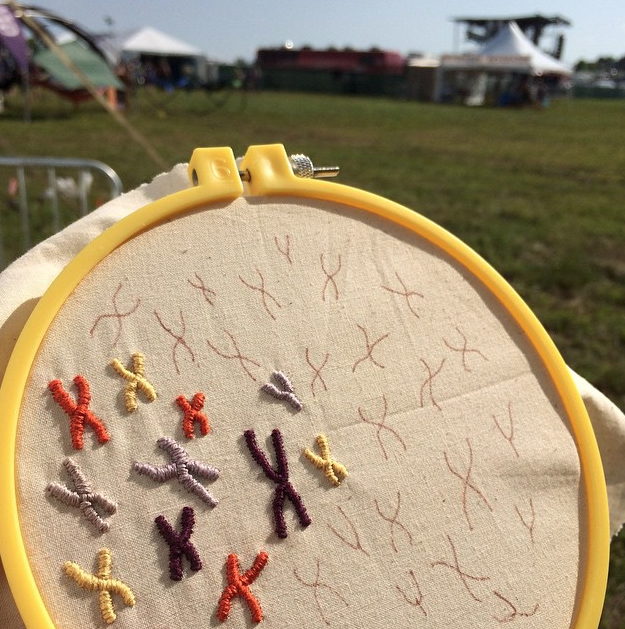This image captures a detailed close-up of a vibrant and colorful embroidery project, taken outdoors on a clear and sunny day at a festival-like gathering. The focal point is a round yellow plastic embroidery hoop holding a tan or light cream linen fabric. The embroidery features X and Y shapes filled with yarn in various hues including red, yellow, burgundy, and different shades of purple. Some shapes are half-completed or outlined in pencil, suggesting the start of a complex design which appears to represent chromosomes. 

The immediate background, slightly blurred, reveals a large grassy field, enhancing the setting's open-air feel. Toward the top of the picture, there are multiple pop-up tents in blue and other shades, indicating a busy fair or festival environment, although no specific details or people are discernible. The overall scene brings a sense of meticulous craftsmanship set against the lively and bustling atmosphere of an outdoor event.